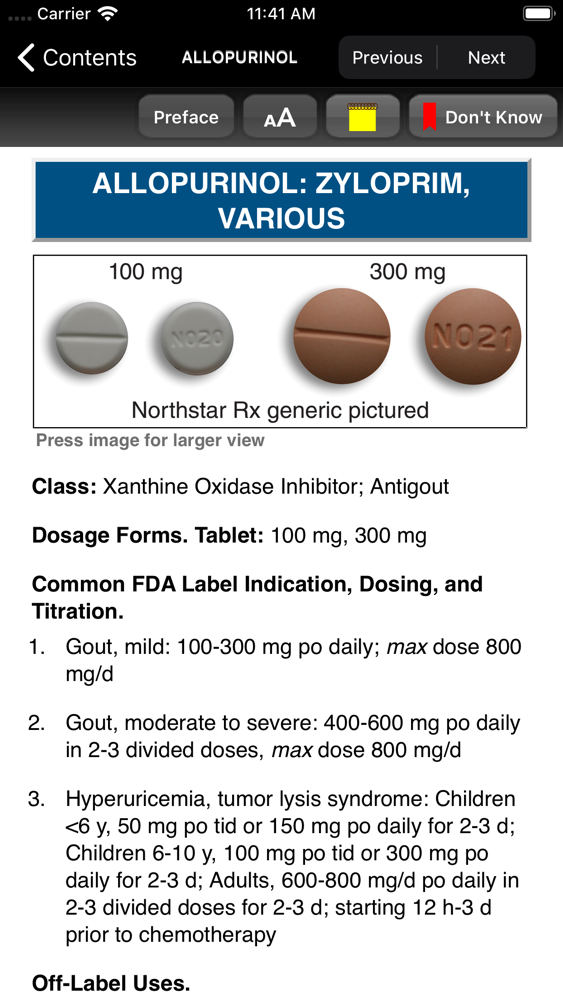Screenshot of a Medical Information Website on Allopurinol

This image is a screenshot from a website with a black header containing white text. On the top left corner, the word "Carrier" is displayed next to a Wi-Fi signal icon. Centrally located is the time "11:41 AM." To the right, a battery icon is shown depleting. Below the header, a navigation bar features a left arrow icon labeled "Contents" along with buttons for "Previous" and "Next."

The main content begins with the title "Allopurinol" in capital letters. This is followed by a "Preface" section, with two buttons featuring letter 'A's—one smaller and one larger—to adjust text size. A yellow notepad icon labeled "Don't Know" and a red ribbon icon are also present.

Underneath this section, the background switches to white with a prominent blue banner that reads "Allopurinol: Zyloprim." Directly beneath, the word "VARIOUS" is displayed in all caps. A thin line creates a rectangle highlighting the visual depiction of Allopurinol tablets. Inside this rectangle, there are images of four tablets: two gray 100 mg pills and two larger brown 300 mg pills. Below this is the label "NorthStar Rx Generic Pictured," followed by the prompt "Press Image for a Larger View."

The medical information provided at the bottom covers classifications, doses, forms, and the common FDA label indications, including usage for "Gout" and "Hyperuricemia." It also mentions "Off-Label Uses."